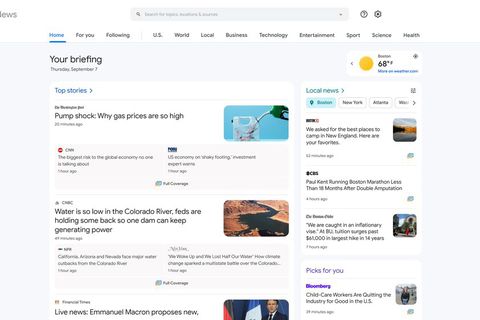In the upper-left corner of the image, the word "LEWS" is displayed in black text against a very low-resolution, pixelated background. Across the center of the image on the same horizontal line as "LEWS," there is a prominent search bar. Following the search bar, to the right, are two small icons, which appear to represent "Settings" and possibly a "Help" or "Question mark" option.

Below this line is a horizontal navigation bar featuring a series of tabs. The tabs, depicted in black text on a white background, are labeled: "Home," "For You," "Following," "US," "World," "Local," "Business," "Technology," "Entertainment," "Sports," "Science," and "Health." The "Home" tab is currently selected.

Underneath this navigation bar, the page presents a header indicating "Your Briefing" and the date "Sunday, September 7th." 

The section titled "Top Stories" follows, featuring several news headlines in a list format:
1. "Pump Shock: Why Gas Prices Are So High" from CNN.
2. A partially visible headline mentioning the global economy with the phrase, "the bigger something to the geo-economy, no one is bulking," though it appears incomplete.
3. "US Economy on Shaky Footing."
4. "Water Is So Low in the Colorado River, Feds Are Holding Some Back, So One Dam Can Keep Generating Power."

Further down, a segment labeled "Live News" features the beginning of another story: "Emerald Macon proposes new," but the text abruptly cuts off.

The overall presentation and clarity of the page are compromised by the very poor resolution, making finer details difficult to discern.